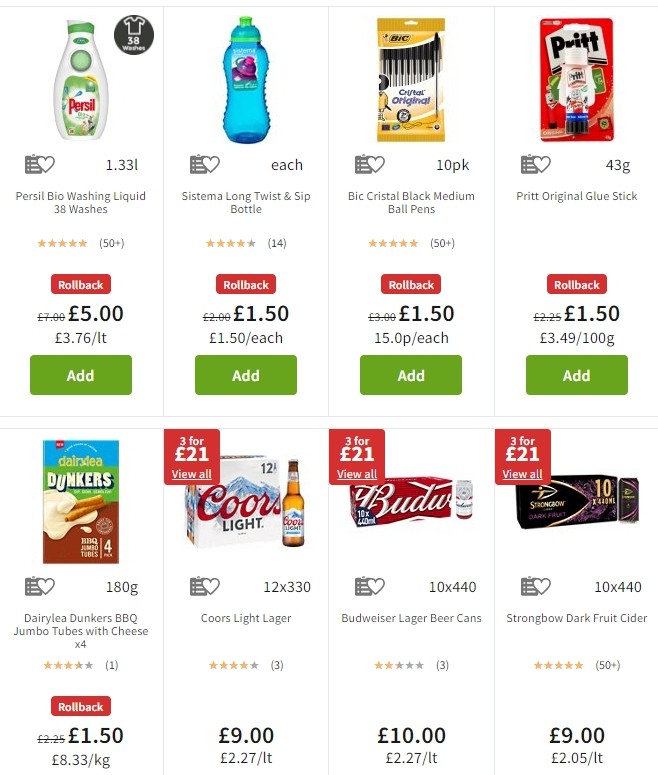This image is a detailed screenshot of a British grocery website. The site interface prominently displays two rows of products, each showing four items in a grid layout. For each product, the interface provides a star rating, the price, and a green "Add" button to facilitate adding items to the shopping cart. 

On the top row, the first product is a bottle of Persil Bio Washing Liquid priced at £5.00. Next to it is a Sistema Long Twist 'n' Sip Bottle, listed at a significantly higher £150.00. Following this is a 10-pack of Bic Ballpoint Pens, costing £1.50, and a Pritt Original Glue Stick, also priced at £1.50. All the items in this row feature red "Roll Back" stickers with white text.

The bottom row showcases a variety of food and beverage items. These include Dunker's Barbecue Jumbo Tubes with Cheese, Coors Light beer, Budweiser, and Strongbow Dark Fruit Cider.

Each product on display includes clearly visible star ratings and prices, providing customers with essential information at a glance, along with the convenient "Add" button to streamline the shopping experience.